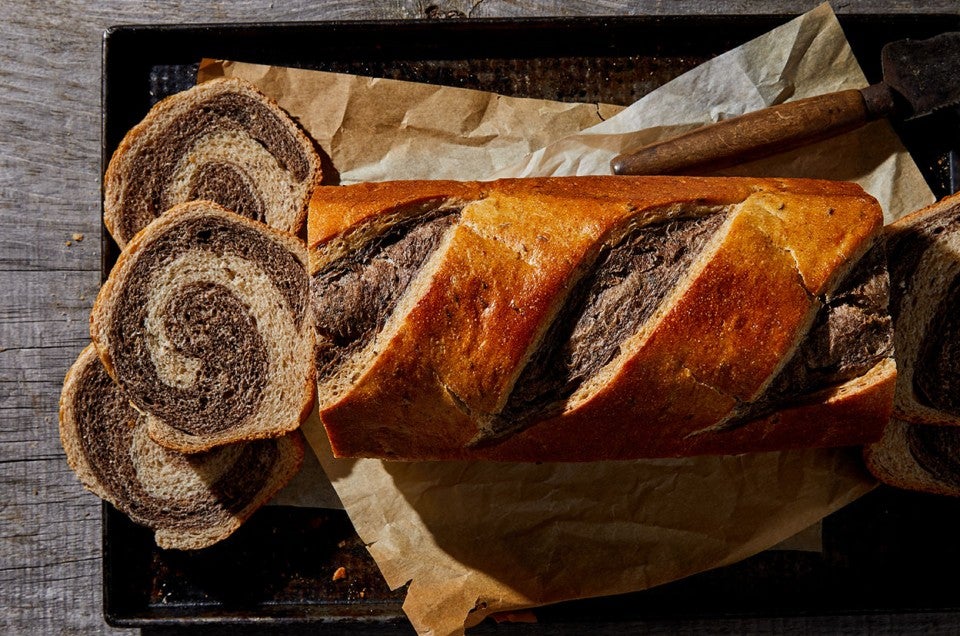This is an aerial photograph of a marble rye loaf of bread, artfully arranged on a dark, blackened baking tray lined with parchment paper. The loaf, which shows a rich interplay of brown and dark brown swirls, reminiscent of a cinnamon roll pattern, has been partially sliced. Three of these slices are facing upwards, revealing the intricate marbled design. Crumbs are scattered both on the baking tray and the surface of the table below. In the upper right-hand corner of the tray lies a serrated knife with a wooden handle, its blade appearing slightly rusted and unpolished. Another serrated piece of bread, partially out of the frame, hints at additional slices. The baking tray, with ventilation holes, rests on a wooden surface that displays a mix of gray and brown hues, border framing 10% of the left side of the picture.